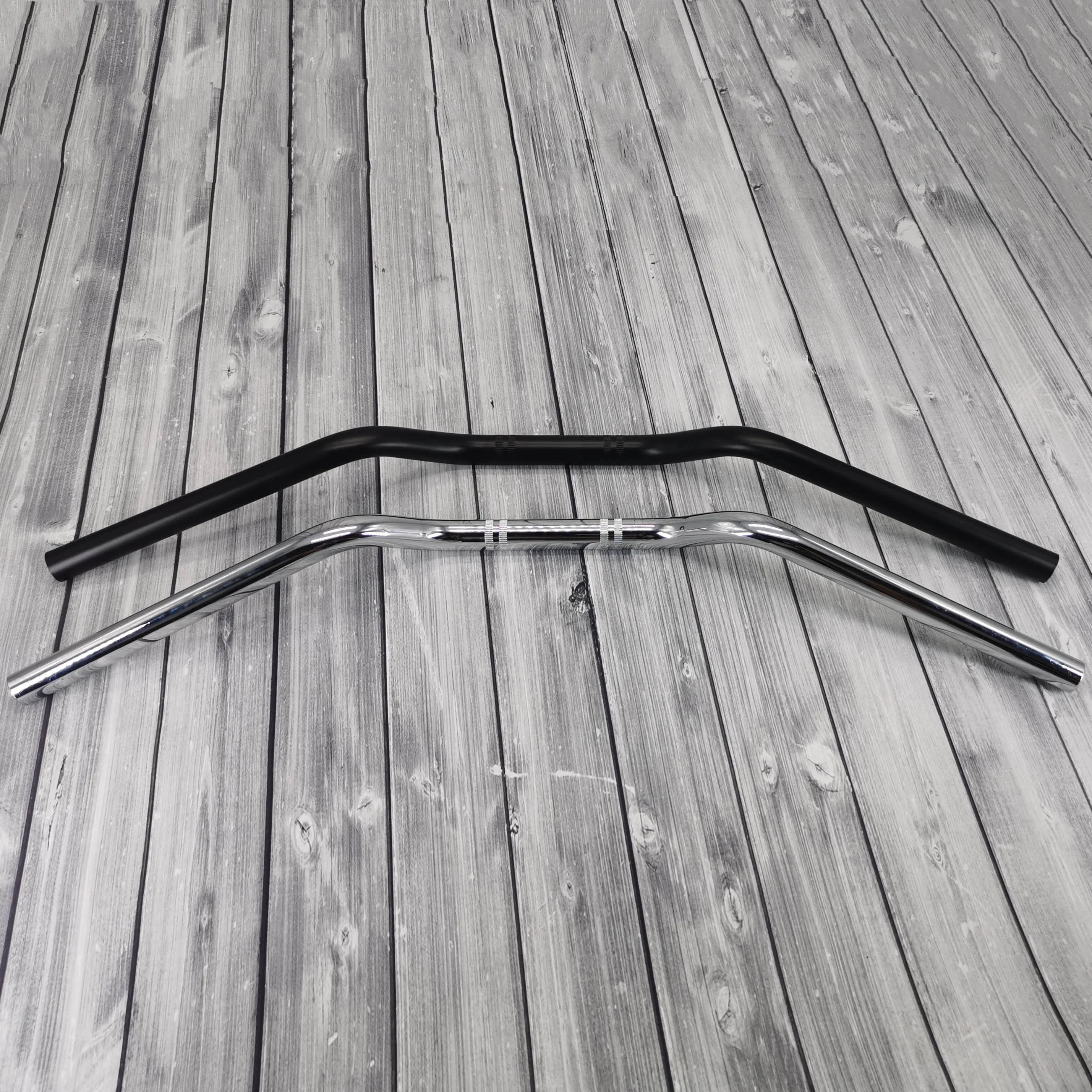The image is a detailed product photograph taken from an aerial viewpoint, showcasing two distinct metal bars laid side by side on a distressed gray hardwood floor. The floor consists of horizontally running, slightly knotty wood planks that are 2 to 3 inches wide. The top bar appears to be about 18 inches long and has a matte black finish. It starts straight, then curves down slightly, rises up again, and dips once more, forming a subtle M shape. Underneath this black bar, there is a shiny, silver-colored bar also bent in a similar M shape. Both bars have distinctive vertical white lines: the black bar has two white lines near the middle, and approximately three inches to the left are another set of vertical white lines. The product's reflective surfaces highlight its metallic texture, emphasizing the contrast between the matte black and shiny silver finishes.